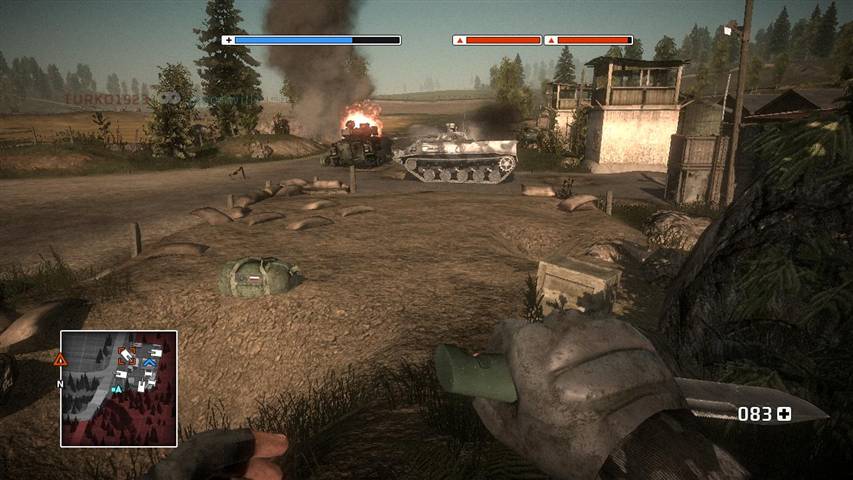The image depicts a dramatic scene from a computer game set in a war-torn environment. In the background, an armored vehicle appears to have been struck, while another intact armored vehicle stands nearby to its right. To the right side of the image, lookout towers and various dwellings are visible, suggesting a fortified base. The ground is littered with boxes and supplies, hinting at ongoing operations or recent conflict.

Flanking the sides of the image are tall trees, adding a sense of depth and framing the scene against a bluish-gray sky, which conveys a somber, overcast atmosphere. In the immediate foreground, the player's hands are shown in first-person perspective: the right hand, gloved and holding a knife, and the left hand wearing a fingerless glove, ready for action.

To the left of the screen, a small square inset provides a night-vision view of the same scene, offering an alternative visual mode to aid in strategic decisions. This detailed depiction serves as a setup for planning an attack on the fortified base, blending tactical gameplay elements with immersive visual storytelling.